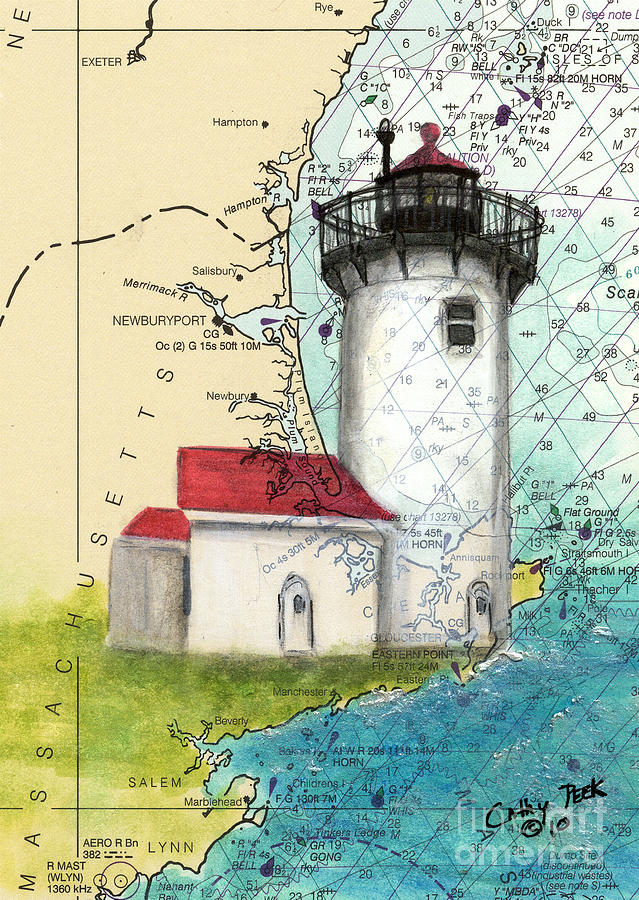The image is a detailed artistic rendering of a white lighthouse with a red roof, superimposed over a map of the eastern coastline of Massachusetts, focusing on several prominent towns and cities such as Rye, Hampton, Salisbury, Merrimack, Newburyport, Manchester, Beverly, Marblehead, Salem, and Lynn. The lighthouse is painted with a smaller house attached to its side, which has a red roof, a single door, and no windows. The lighthouse itself features a single door, a single window, and a traditional balcony, topped with metal grating. The map beneath is relatively featureless except for land, water, and city names, along with lines and number markings indicating navigational information on the right-hand side. The artist’s signature, Cathy Peak, covers a portion of the text "Fine Art America" in the lower right corner. The overall color scheme includes blue, white, red, black, tan, and green.